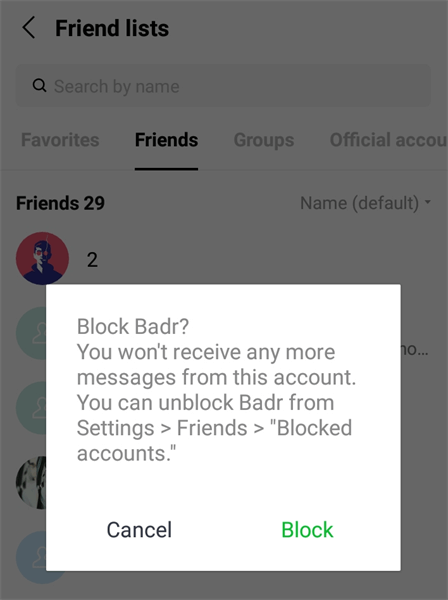**Image Caption:**

The image showcases a user interface from a social networking website. A translucent gray overlay is spread across the screen, dimming the underlying content. Central to the scene is a prominent white pop-up box with a message asking, "Block Badr?" This message indicates that blocking will stop any future messages from this account. Options presented in the pop-up include a gray "Cancel" button and a green "Block" button, urging the user to decide their next course of action.

Behind the pop-up, the partially obscured friends list interface can be observed. The section offers options such as 'Search by Name,' 'Favorites,' 'Friends,' 'Groups,' 'Official Accounts,' as well as displaying a total of 29 friends. Although the gray film and the pop-up obscure some details, it is evident that one friend is mutual with two others, and five friends are visible beneath the overlay.

At the top of the interface, the user's name is displayed along with a dropdown menu, granting access to additional settings. Notably, the user can navigate to 'Settings,' 'Friends,' and 'Blocked Accounts' sections if they want to review or alter their friends or blocked individuals later on. The pop-up highlights "Badr" as the user to potentially block, reminding the user that should they choose to block, they can adjust this decision in the future from the designated settings menu.